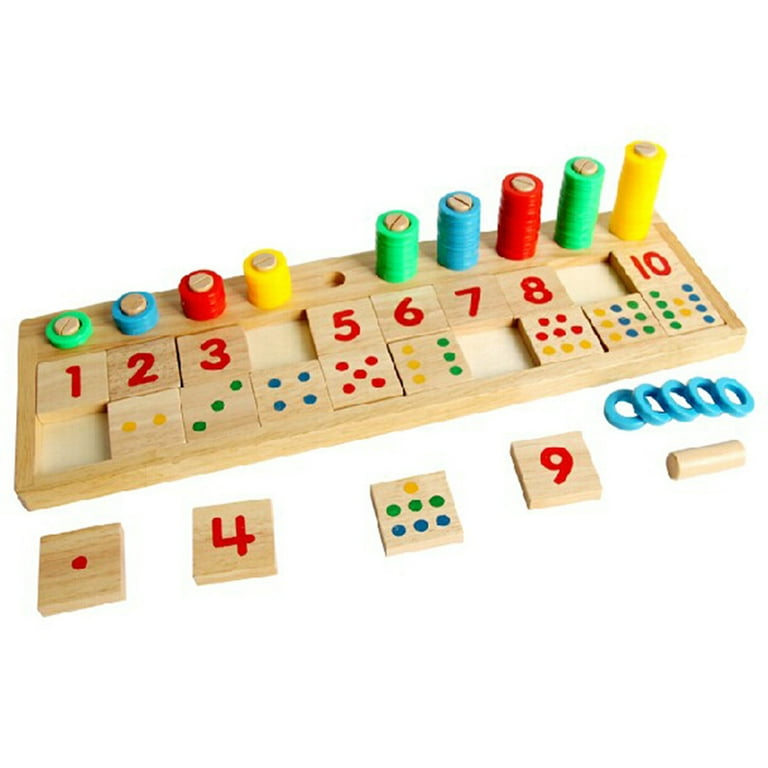The image depicts a child's wooden counting toy set with a beige finish. The toy features 10 pegs at the top, around which colorful plastic rings—ranging from green, blue, red, to yellow—can be placed. Below the pegs, there are wooden blocks displaying numbers from 1 to 10 in red. Each numbered block has a corresponding block with dice dots ranging from 1 to 10 dots: one dot is red, two dots are yellow, three dots are green, four dots are blue, five dots are red again, six dots combine yellow and green, and additional colors form combinations up to 10 dots. Notably, the blocks corresponding to the numbers/ dice faces for 1, 4, 7, and 9 are missing. The toy appears to be designed to help children learn to count and recognize numbers and dice faces, all while engaging with colorful visual aids. The image seems to be a close-up digital screenshot of this educational toy.